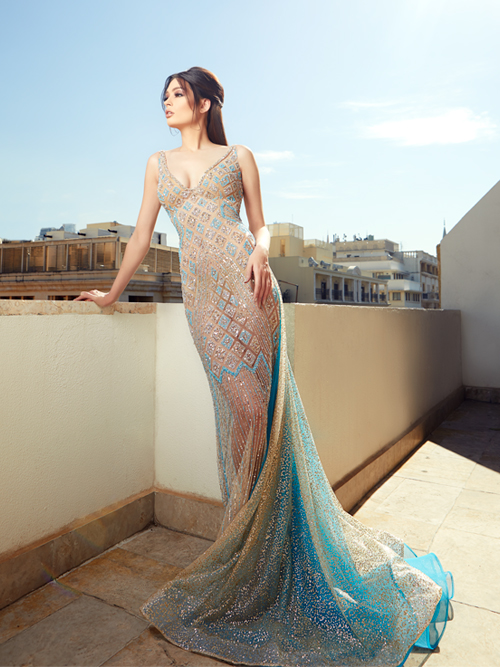In this hyper-realistic and modern image, a woman, presumably a model, is posing on a rooftop terrace against a waist-high stone guardrail. She is dressed in a flowing and elegant, somewhat transparent dress adorned with blue and gold diamond patterns. The dress showcases a gradient from transparent to a more opaque, pleasant light blue towards the skirt area, resembling an ocean color. The dress extends past her feet and features a V-cut design, giving it a mermaid-style appearance. She has brown hair and is captured in a profile shot as she leans against the guardrail with her right hand, looking off into the distance to the left. The background reveals a clear, sunny day with a blue sky and several tan and light brown buildings, indicating that the setting could be in a city center.